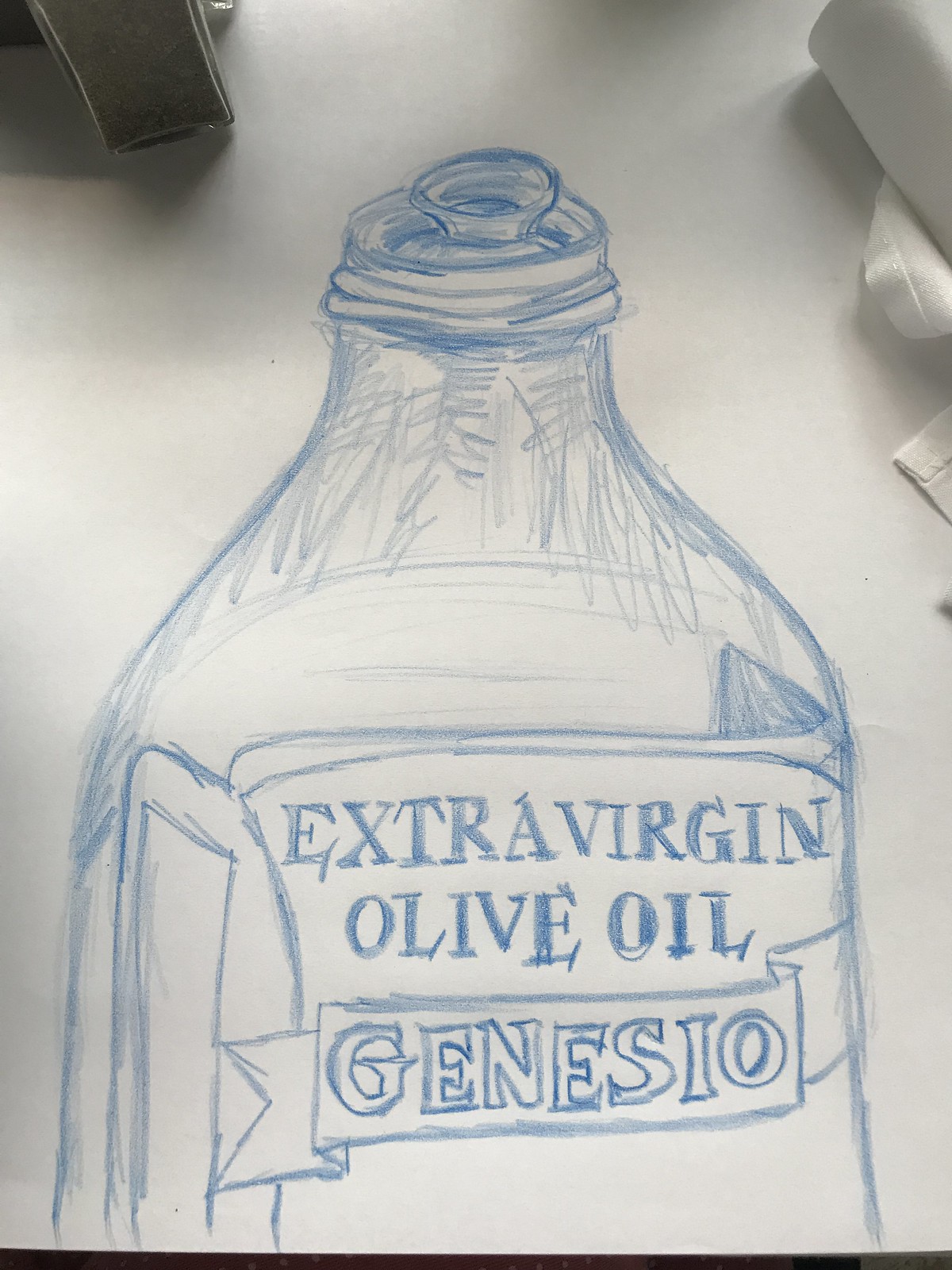This is a detailed blue pencil drawing on white paper, depicting the upper half of a bottle of extra virgin olive oil. The bottle is prominently featured in the center of the composition. The bottle's opening is detailed with a plastic lip and pour spout. Below the opening, the label reads "Extra Virgin" with "Olive Oil" beneath it and the brand name "Genesio" elegantly displayed on a ribbon. The illustration also includes subtle shading near the top and left side of the bottle, suggesting depth and contour. In the upper left corner, there is an indeterminate brown object, while the upper right corner features a rolled-up white cloth napkin, adding elements of context to the sketch.